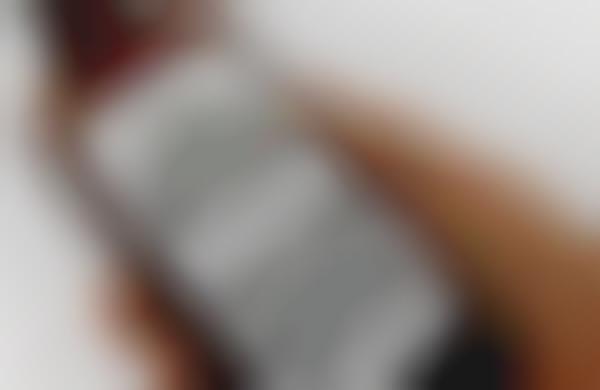The image is notably blurry, making detailed identification challenging. It features a rectangle with a white, somewhat indistinct upper right corner, transitioning into a brownish hue that runs down the center. Overlaid on this brownish strip is a white or possibly silver, curved rectangle, suggesting the outline of a device such as a cell phone. This central figure is flanked by a continuous white or grayish blurry background. The brownish-red and almost black colors suggest that a Caucasian hand might be holding the cell phone, which lacks any visible text on its screen. Despite the severe blurriness obscuring many details, the general consensus leans towards interpreting the image as depicting a hand holding a cell phone, set against a pale background.